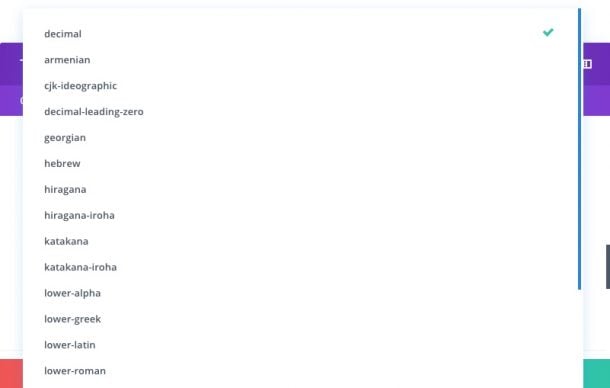This image is a cropped screenshot of a pop-up box displaying a vertical list of search options or selectable items. The first item in the list, labeled "Decimal," is highlighted with a green checkmark indicating it is selected. Below "Decimal," the list includes various other options such as "Armenian," "CKG Ideographic," "Decimal Leading Zero," "Georgian," "Hebrew," "Hiragana," "Hiragana Aroha," "Katakana," "Katakana Aroha," "Lower Alpha," "Lower Greek," "Lower Latin," and "Lower Roman," before the screenshot cuts off.

On the right side of the pop-up box, a blue scroll bar is visible, positioned at the top, indicating more options are available to scroll through. Surrounding the pop-up box, the screen is segmented into different color sections: purple at the top left and right corners, white in the central background area, red in the bottom right, and green in the bottom left. The pop-up box itself stands out against these multicolored sections, emphasizing the list of selectable items.